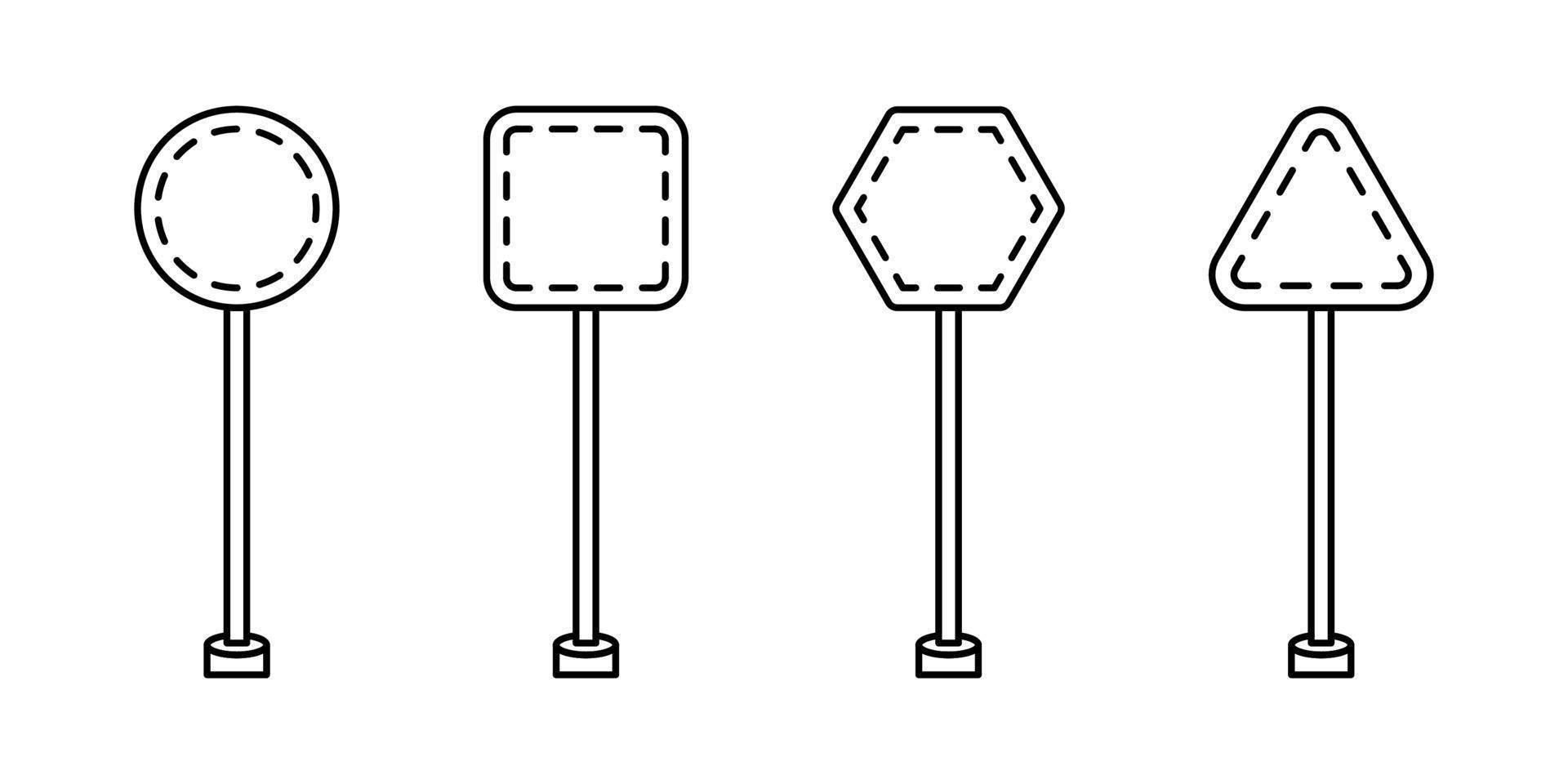The image appears to be a series of computer-generated design prototypes that resemble street signs, arranged from left to right. The designs, all in black and white, feature different geometric shapes: a circle, a square, a hexagon, and a triangle. Each sign is intricately detailed with dotted lines inside that correspond to the perimeter of the respective shape. Furthermore, the composition of each design includes a top section with the primary shape, a thinner middle section, and a cylindrical base at the bottom.